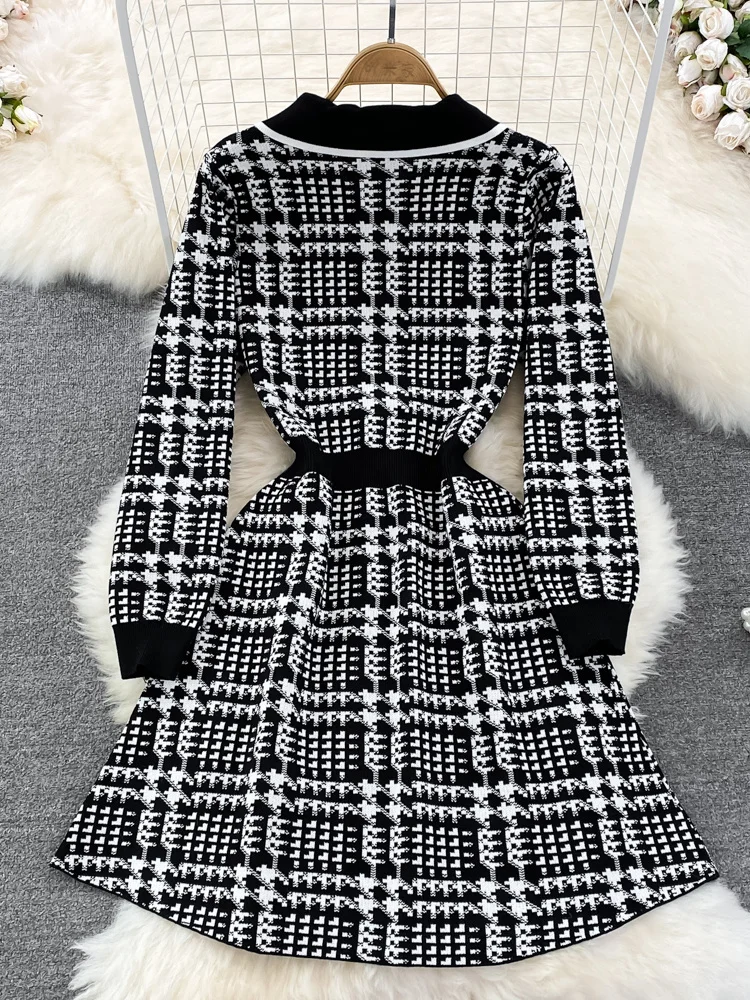This photo showcases a long sleeve dress hung on a brown wooden hanger. The dress, which appears to be a product display, features a black and white checkered or pixelated pattern that resembles houndstooth, creating a textured and almost 3D effect. It has a solid black straight collar, black cuffs, and a cinched waist made of stretchy black knit material. The dress is medium length with loose sleeves. The setting reveals the dress partially hanging on a rack and draped over a chair covered in white faux fur. A white sheepskin-like rug is seen underneath and surrounding the dress, adding a contrast to the overall presentation.